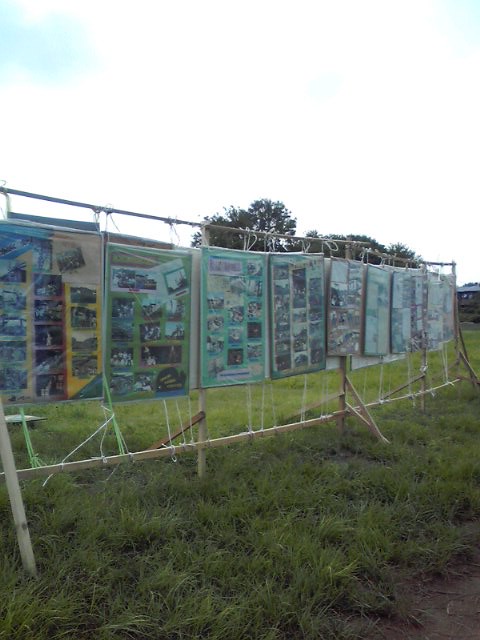The photograph depicts a series of poster boards suspended by strings on a wooden frame-like structure situated in a grassy field. There are roughly ten poster boards, each filled with numerous photos arranged in a vertical alignment, possibly some being four by six inches in size. The contents of the pictures are not distinctly visible due to the plastic covering and distance, though glimpses suggest they might depict people or teams, with some posters potentially containing text. The scene is set against a backdrop of tall, uncut grass, with trees visible in the distance and patches of blue sky peeking through the mostly cloudy atmosphere. The entirety of the photo boards stretches both horizontally across the image and at an angle from the foreground to the background, suggesting a comprehensive visual display.